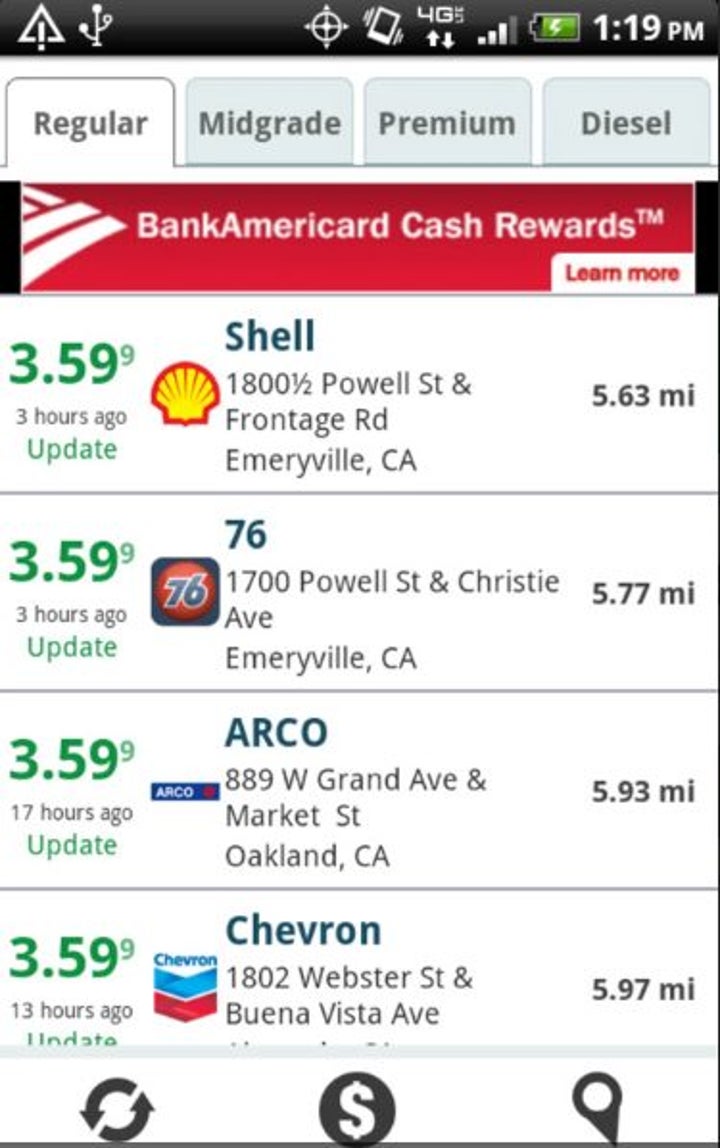A screenshot displays a mobile app interface used for searching and comparing gas prices. At the top of the screen, standard phone indicators show a battery percentage and a time of 1:19 pm. Below this, the app allows users to choose gas types: Regular, Mid-Grade, Premium, and Diesel. An advertisement for Bank of America Cash Rewards is featured prominently.

The main section lists various gas stations starting with Shell at the top. The Shell listing includes its logo, address, and gas price of $3.59 per gallon, presented in green text. It also indicates a distance of 5.63 miles from the user's location, shown in dark gray text. Following Shell, the 76 gas station is similarly presented, with the same price and a distance of 5.77 miles.

Also listed are ARCO and Chevron stations, each displaying logos, addresses, and the price $3.59 in green text. Distances for these stations are not specified but are likely listed in the same dark gray below the prices. 

At the bottom of the screen, there are three icons for additional functionalities: a refresh icon, a money icon, and a location icon, presumably for refreshing the listings, financial details, and location services respectively.